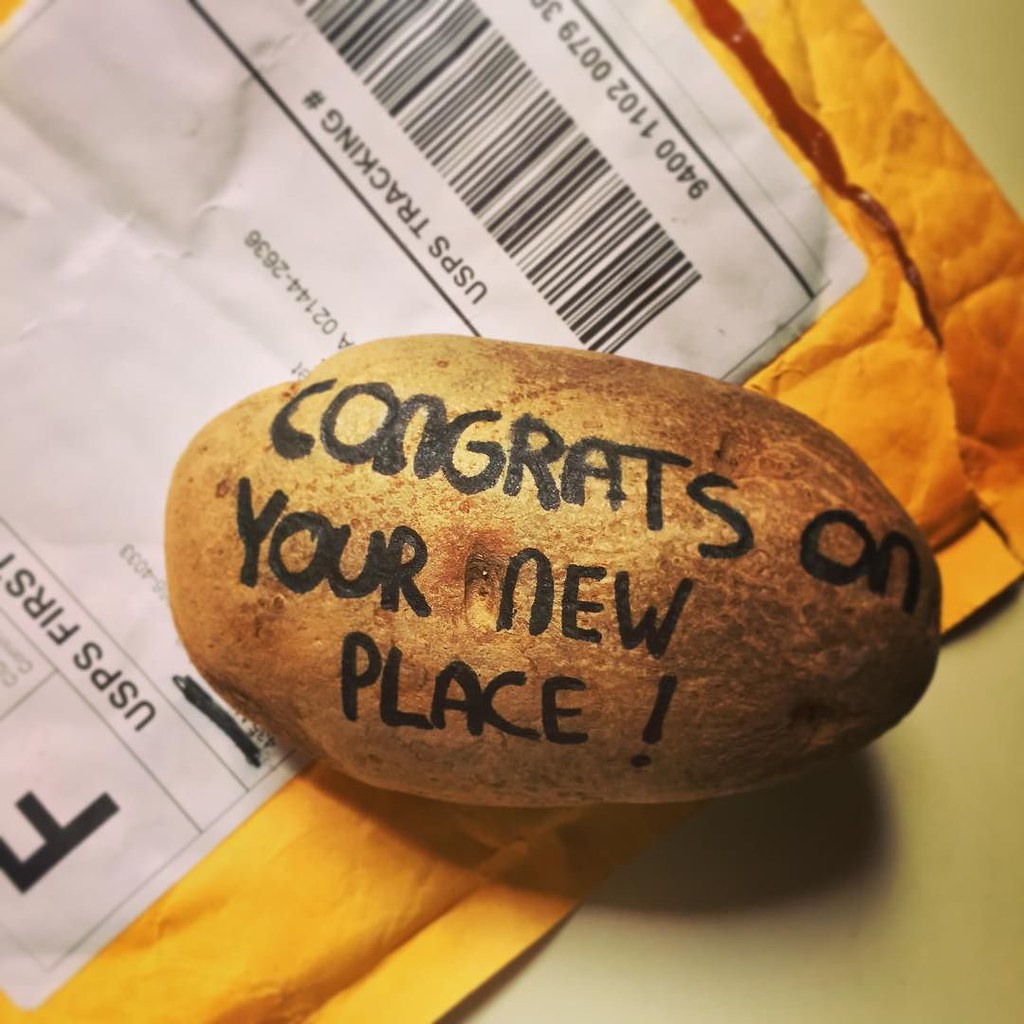In the image, a plain russet potato sits on a torn, yellow manila envelope, with the remnants of a USPS first-class mailing label visible. The text "Congrats on your new place!" is handwritten in black sharpie directly on the potato. The envelope underneath, set on a white countertop, features a partially visible USPS tracking barcode and the number A02144-2636. The name on the label has been crossed out, suggesting some privacy protection. The potato, centered in the image, adds a whimsical and unexpected element to the scene.